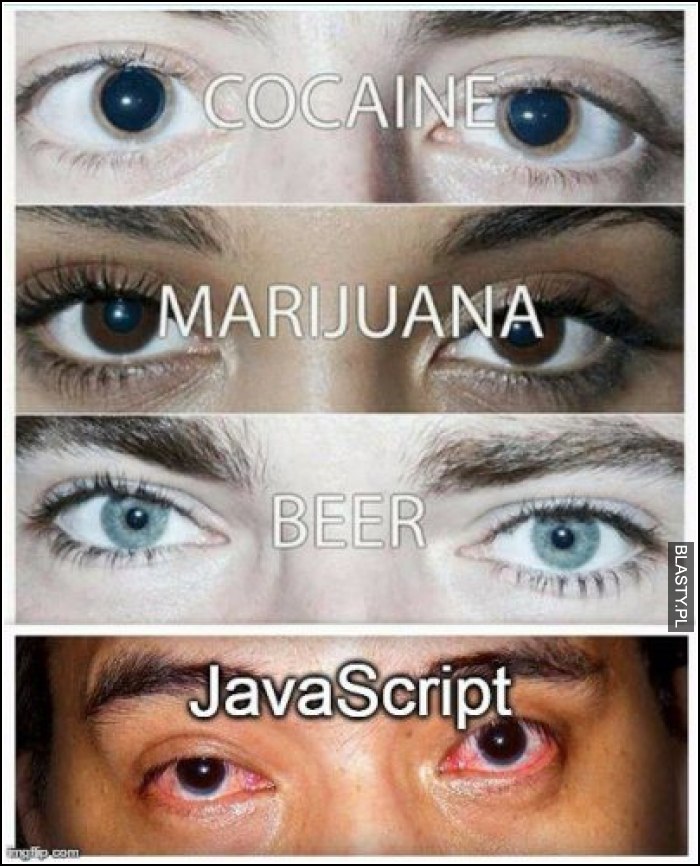The poster humorously depicts the influence of various substances through close-up images of four sets of eyes arranged in a single column. The first set at the top features a white person with normal-looking brown eyes under the label "COCAINE" written in white capital letters across the eyes. The second set belongs to a dark-skinned individual with brown eyes labeled "MARIJUANA" in white capital letters. The third image shows a white person with blue eyes and brown eyebrows, with the word "BEER" displayed in white capitals across the bridge of the nose. The final and most striking set of eyes, belonging to a darker-skinned person, is noticeably bloodshot and marked with the term "JAVA SCRIPT" in white capital letters across the forehead, suggesting the intense toll of working with JavaScript compared to the effects of drugs or alcohol.